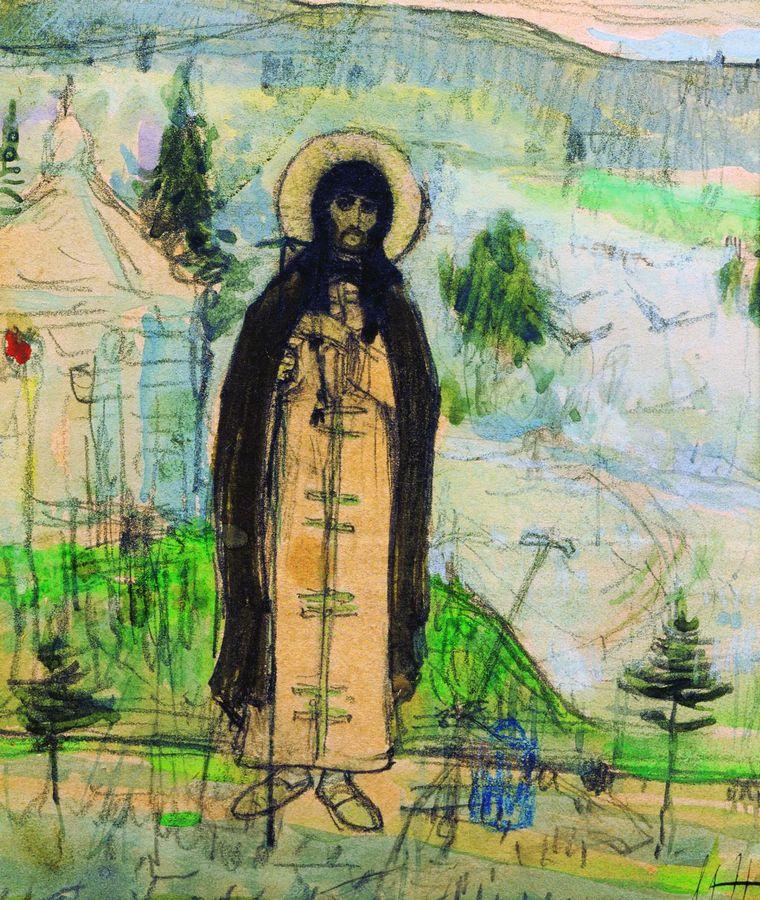The image appears to be a child-like crayon or colored pencil drawing that prominently features a central figure resembling Jesus, characterized by long hair, a beard, and a halo around his head. The figure is dressed in a peach-colored robe that reaches down to the ankles, with indications of additional cloth or a long coat, and wears light yellow shoes. The background is a whimsical landscape with green hills, a few rudimentary trees, and what looks like a teepee-style building or perhaps a small church. The sky above is a mix of peach and blue hues. The ground is depicted with blue and green grass, and small, not-to-scale trees that hardly reach the figure's shins. In the lower part of the image, near Jesus's left side, there's an indeterminate blue object. The overall color scheme centers on greens, blues, yellows, and peaches, giving the scene a vibrant yet elementary feel, reminiscent of a child's imaginative drawing.